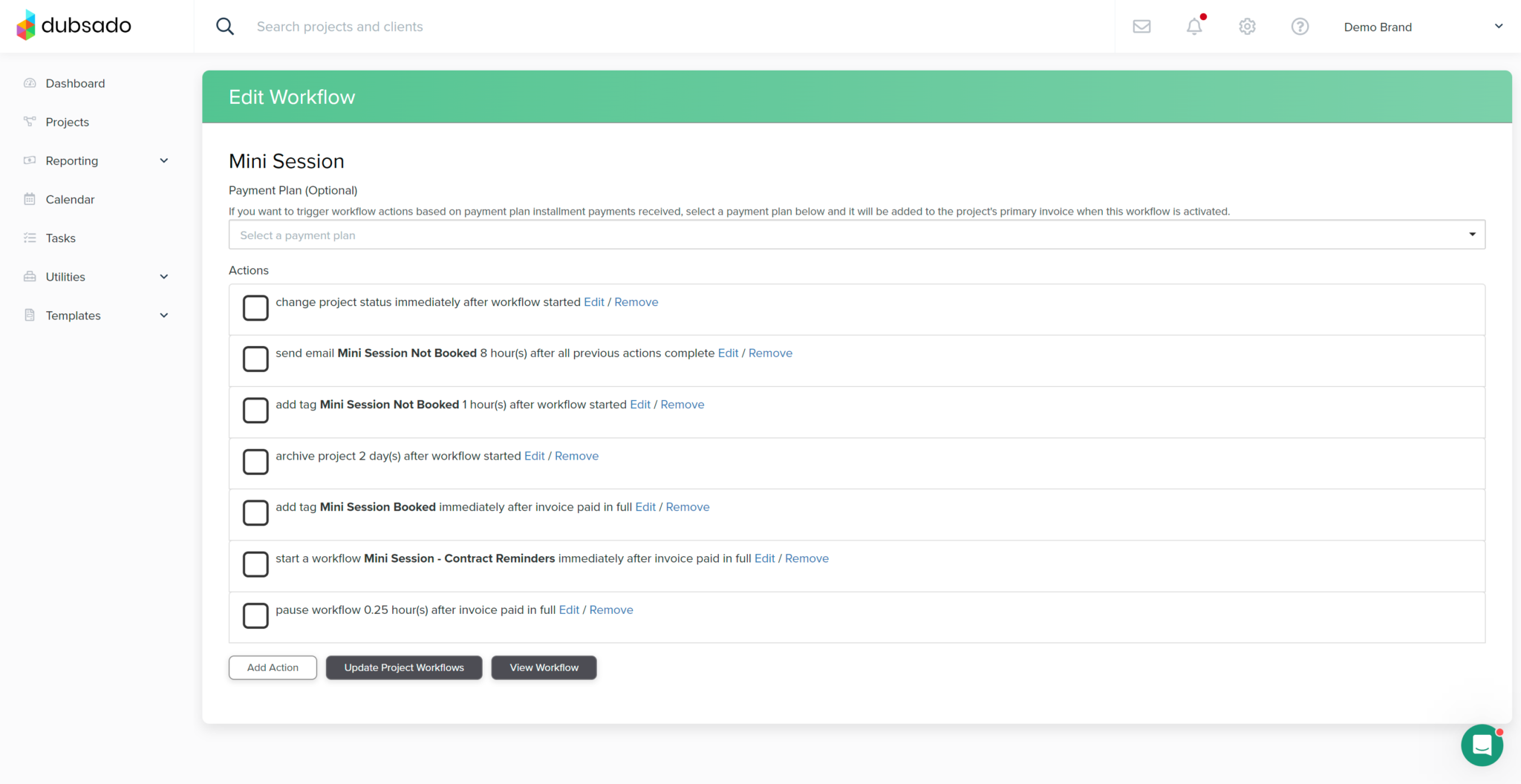Here's a refined and detailed descriptive caption for the image:

---

The image is a screenshot of a project management application named "Dubsado." In the upper left corner, there is a logo consisting of a red, yellow, green, and blue cube adjacent to the "Dubsado" text. Next to the logo are a search bar, a mail icon, a notifications bell, a settings cogwheel, and a question mark icon for help. The upper right corner displays "Demo Brand."

On the left side, a vertical gray sidebar includes selectable options: Dashboard, Projects, Reporting, Calendar, Task, Utilities, and Templates.

To the right, a prominent green banner with white text reads "Edit Workflow." Below the banner, a white section contains black text beginning with "Mini Session, Payment Plan Option." The text instructs users to trigger workflow actions based on payment plan installment payments received. Users can select a payment plan to add it to the project's primary invoice and activate the workflow.

Below the instructions, there are several workflow actions listed:
1. Save project status immediately after workflow starts (with Edit and Remove options).
2. Send email "Mini Session Not Booked," eight hours after all previous actions are completed.
3. Add tag "Mini Session Not Booked," one hour after the workflow starts.
4. Archive project two days after the workflow starts.
5. Add tag "Mini Session Booked," immediately after the invoice is paid in full.
6. Send "Mini Session Contact Reminders" immediately after the invoice is paid in full.
7. Pause the workflow 0.25 hours after the invoice is paid in full.

At the bottom, options include "Add Action," "Update Project Workflows," and "View Workflow."